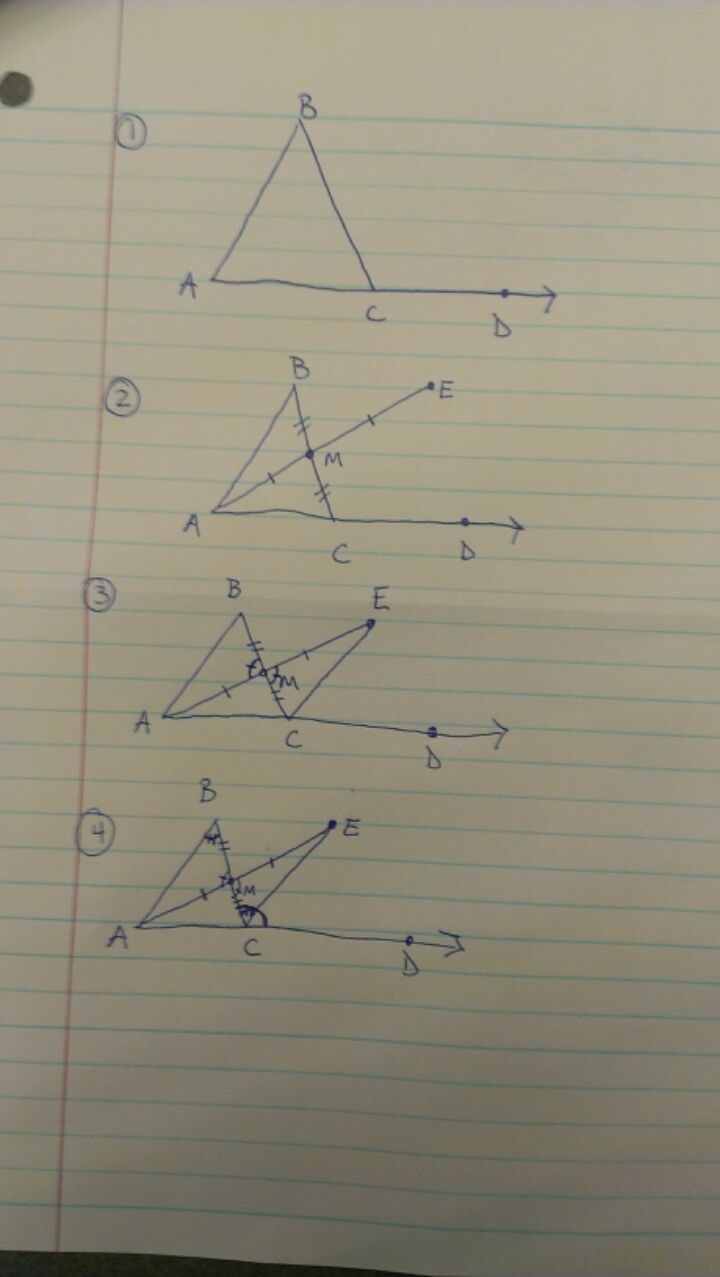This photograph captures what appears to be a student's geometry homework resting on a desk. The homework features four geometric figures, each building progressively on the previous one. 

1. The first figure is a triangle with vertices labeled A, B, and C. Additional point D lies on the extension of the side BC and is marked with an arrow pointing to the right.
2. The second figure closely resembles the first but introduces an additional line segment. This line extends from vertex A, intersects the side BC, passing through its midpoint, and extends out to a new point labeled E.
3. The third figure builds further by adding another line segment connecting E and C, resulting in a shape that somewhat resembles a bow tie.
4. The fourth and final figure mirrors the third but includes a curved line in the lower right corner above point C, adding complexity to the diagram.

The image is meticulously detailed, showcasing incremental changes through each geometric configuration, reflecting a step-by-step problem-solving approach.